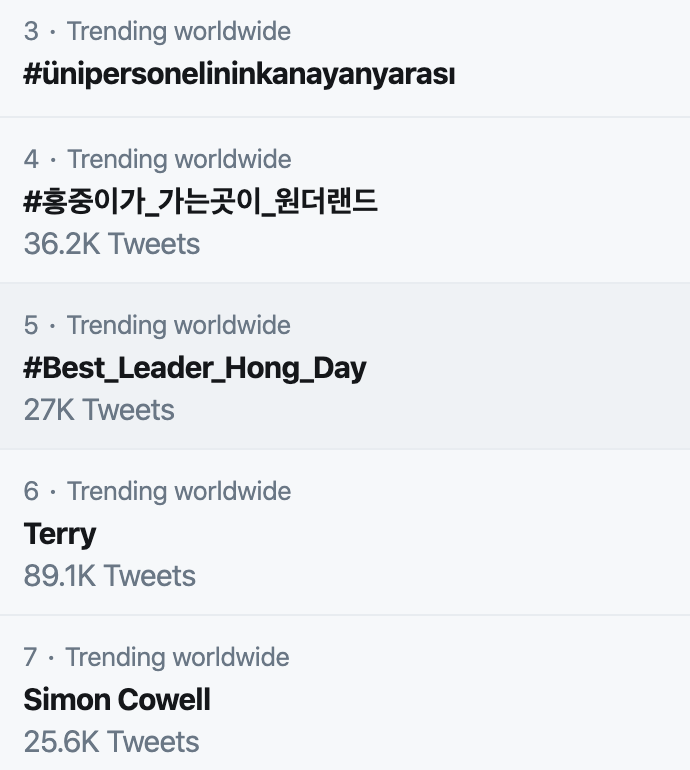The image features a detailed list of worldwide trending topics displayed against a light gray background. 

At the top, in a light gray color, the ranking begins with "3 - Trending Worldwide," followed by the black hashtag "#UNIPERSONELININKANAYANYARSI."

Following this is the number "4 - Trending Worldwide," written in Asian kanji characters, indicating it's not easily interpretable. This entry has accrued 36.2K tweets, noted just below it.

Moving down to number "5 - Trending Worldwide," marked by the black hashtag "#BestLeaderHongDay," which has garnered 27K tweets, as stated underneath.

The trend list continues with number "6 - Trending Worldwide," where the word "Terry" appears in black text, reaching 89.1K tweets according to the information provided below.

Finally, the list concludes with number "7 - Trending Worldwide," highlighted by the name "Simon Cowell" in black text, attracting 25.6K tweets as indicated in gray beneath the entry.